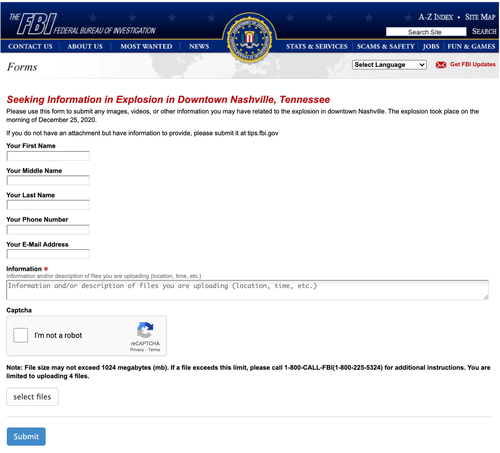The image depicts an official FBI website, identifiable by a blue border at the top. In the left corner, it prominently displays "FBI Federal Bureau of Investigation," while in the far right corner, there is an "A to Z Index." Alongside it are clickable links for a sitemap and a search bar labeled "Search site." To the left, navigation options include "Contact Us," "About Us," "Most Wanted," "News," "Scams and Safety," "Stats and Services," "Jobs," and "Fun and Games," centered around the iconic FBI emblem.

In the main content section, a red alert headline reads "Seeking Information on Explosion in Downtown Nashville, Tennessee," urging users to utilize the provided form to submit any images, videos, or other information related to the explosion that occurred on the morning of December 25, 2020. Users are directed to an alternative submission site, tips.fbi.gov, if they have information without attachments. Below this, a form is laid out with fields for "First Name," "Middle Name," "Last Name," "Phone Number," "Email Address," and an area to enter additional information. There’s a CAPTCHA checkbox labeled "I'm not a robot," followed by an image upload option to attach files and a blue "Submit" button located at the bottom left.